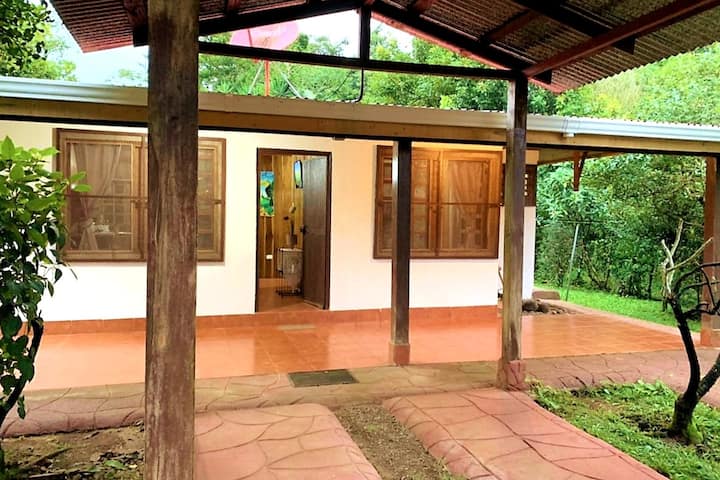The image depicts a small, rectangular, one-level dwelling, possibly a guest house or cabin, located in a tropical or rainforest-like setting. The building features a pristine white stucco facade with wooden-framed windows and a dark brown doorway. In front of the building, the porch boasts columns made of wood supporting a roof, and the floor is covered in shiny terracotta tiles. Extending from the porch area, there are pathways leading to a pavilion with a corrugated metal roof, supported by wooden posts. The pavilion features red stamped concrete platforms interspersed with patches of dirt. Surrounding the structure, vibrant green leaves from nearby trees and bushes enhance the tropical ambiance, and the overall scene appears freshly damp, indicative of a recent rainfall.